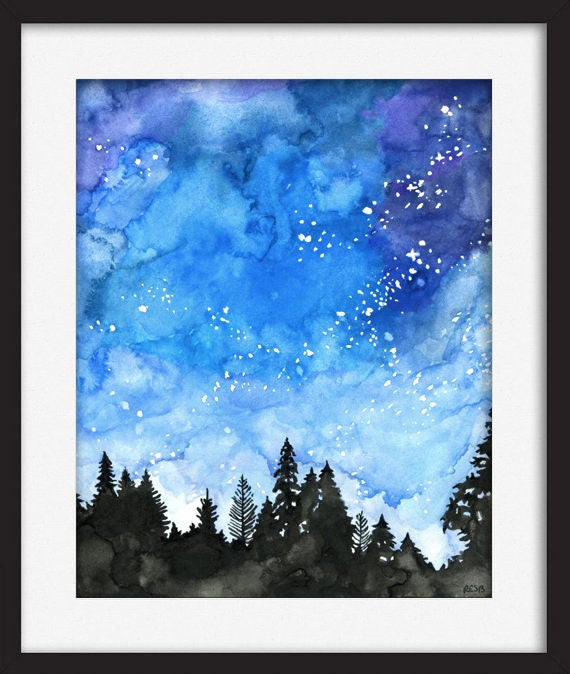The image features a framed painting with a black outer frame and a white inner border that accentuates the artwork. The painting itself is a hyper-realistic depiction of a forest beneath a swirling, dynamic sky. The sky is filled with various shades of blue, gray, and purple, creating a profound and mesmerizing effect. Small white specks, resembling stars or glitter, punctuate the clouds, adding a touch of whimsy to the scene. The forest below consists of various types of trees, including some that appear to be pine and others that have lost their needles, rendered in stark black silhouettes. This creates a dramatic contrast with the vibrant sky above. The bottom of the painting shows the undulating outline of the tree line, giving the impression of a hilly landscape. The painting evokes a sense of mystery and wonder, reminiscent of a starry night in a dense forest.